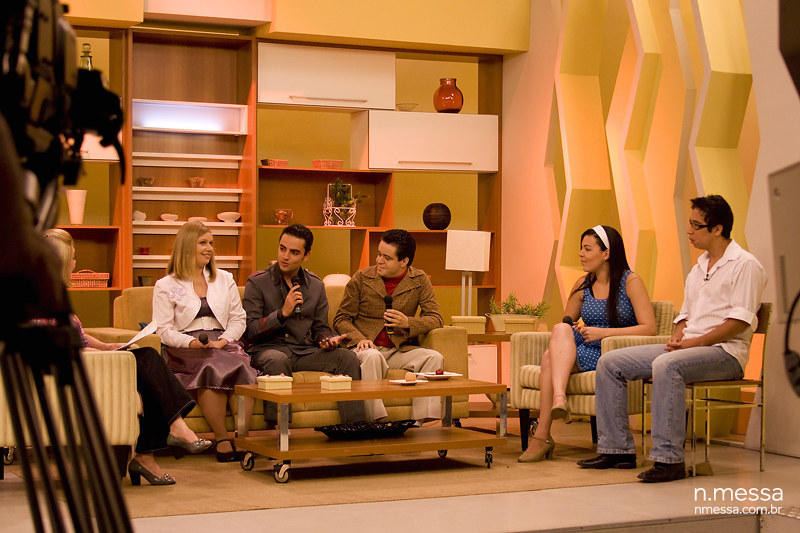The image depicts a retro-style talk show set with six people sitting across a staged faux room. The backdrop features orange and yellow hues mixed with brown shelves that hold various items, such as plates, vases, and knickknacks, contributing to its seventies aesthetic. The seating arrangement includes a small yellow couch with vertical stripes in the center, occupied by three individuals: a woman in a white jacket and purplish skirt on the left, a man in a brown shirt holding a black microphone in the middle, and another man in a brown jacket also holding a black microphone on the right. To the left of the couch, a woman sits in an armchair, dressed in black slacks and appearing to be the host, as she is holding white papers. On the right side of the set, two more people are positioned in chairs: a woman in a blue dress with a white headband holding a microphone, and a man in blue jeans and a white button-up shirt. A coffee table is centrally located in front of the couch, anchoring the setup. The room's walls feature brown geometric shapes and yellow zigzag patterns, reflecting the retro theme.